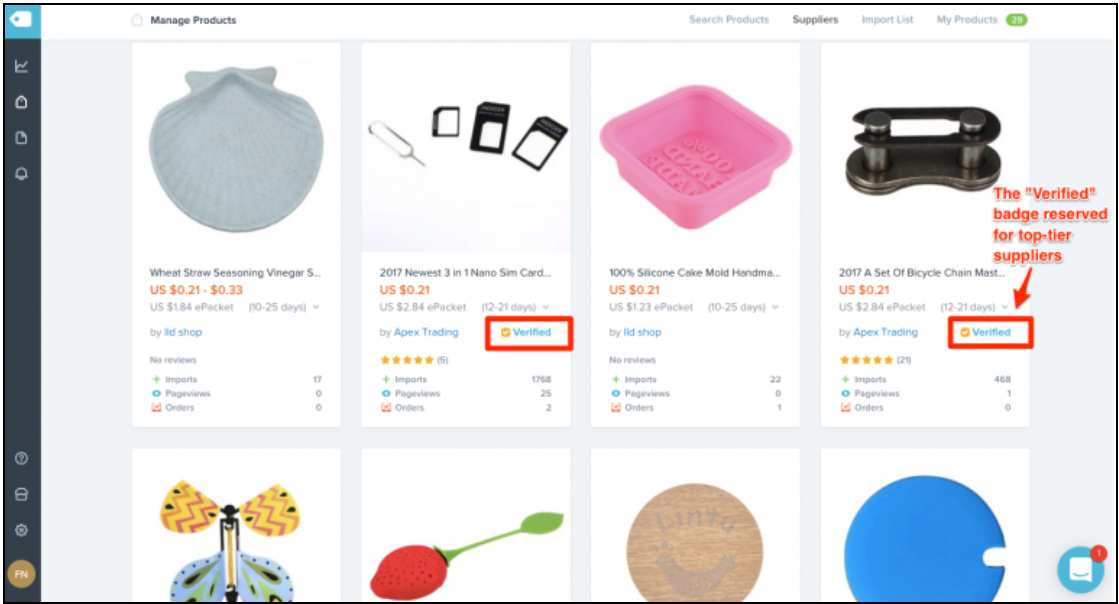The e-commerce website interface showcases a well-organized layout for managing products. In the top left corner, there's an icon resembling a tag, tilted to the left and enclosed in a small blue box. To its right, a bold black text reads "Managed Products." Further right, approaching the center of the screen, there are additional navigation options: "Search Products, Suppliers," which is highlighted in black, "Import Lists," and "My Products." Adjacent to these options is a small green button displaying the number "29."

On the left-hand side, a vertical black toolbar contains various icons, ending with a circular profile icon at the bottom. The main content area is labeled "Managed Products," and immediately below are media images. Eight images are partially visible; four are fully seen while four others are cut off. One of the visible images appears to depict a shell and is titled "Wheat Straw Seasoning Vinegar," complete with pricing information beneath it.

Out of the four fully visible images, two feature a "Verified" badge. This badge is highlighted with a red outline and indicates a distinction reserved for top-tier suppliers.